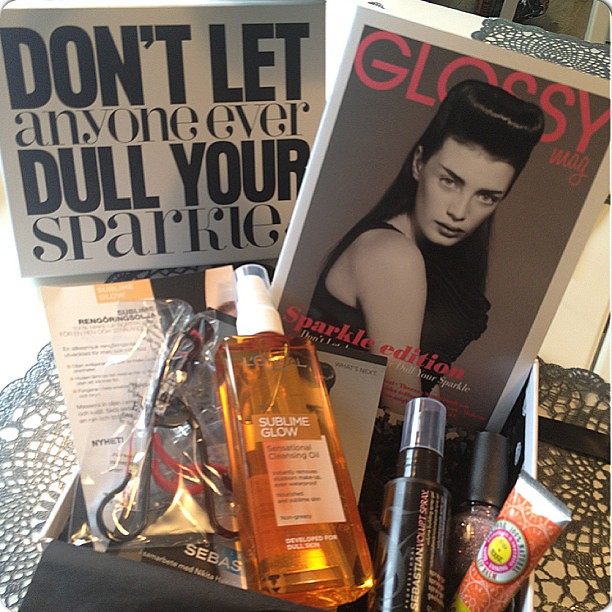The image depicts a detailed assemblage of beauty products presented as part of a subscription box. Dominating the scene is a large rectangular-shaped spray bottle filled with orange liquid and labeled "Sublime Glow" conditioning oil. The box features multiple other beauty items, including additional spray bottles, a nail polish, and an eyelash curler. Overlaying some of these products is a magazine titled "Glossy Mag Sparkle Edition," which showcases a black-and-white photo of a woman with jet black hair styled dramatically. Adjacent to the magazine, a sign boldly declares, "Don't Let Anyone Ever Dull Your Sparkle." This affirming message and the glossy visual elements collectively highlight an emphasis on beauty and self-expression.